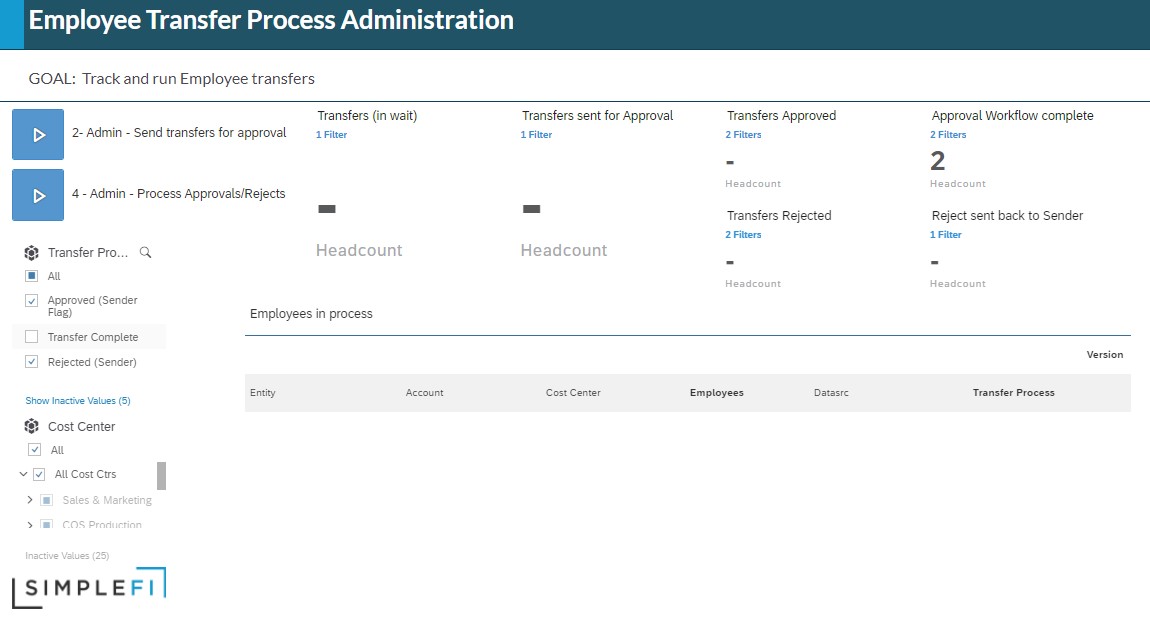The image depicts a webpage dedicated to the Employee Transfer Process Administration. At the top, there is a dark gray banner with a subtle blue tinge in the top left corner. Positioned prominently in white text on the banner are the words "Employee Transfer Process Administration."

Below this banner lies a predominantly white background with another blue banner bearing the text: "Goal: Track and Run Employee Transfers." Progressing further down, there are two prominent blue boxes with white arrows pointing to the right.

The first blue box reads "2-Admin, Send Transfers for Approval," and to the right of it is a horizontal series of steps illustrating the transfer process, which include:
- "Transfers in Wait" with 1 filter
- "Transfers Sent for Approval" with 1 filter
- "Transfers Approved" with 2 filters
- "Approval Workflow Complete" with 2 filters

Returning to the left side, the second blue box, labeled "4-Admin, Process Approvals/Rejects," is followed by two thin black horizontal lines marked "Headcount." Continuing this series horizontally, the steps include:
- "Transfers Rejected" with 2 filters
- "Reject Sent Back to Sender" with 1 filter, also marked "Headcount"

Further down on the left-hand side, beneath the blue boxes, there are various checkmark options related to transfers. At the bottom, a logo resembling the company name "Simplify" is visible.

Overall, the layout is designed to clearly delineate the stages of the employee transfer process, from initiation and approval to rejection and headcount assessment, with a structured and detailed interface to guide administrators.